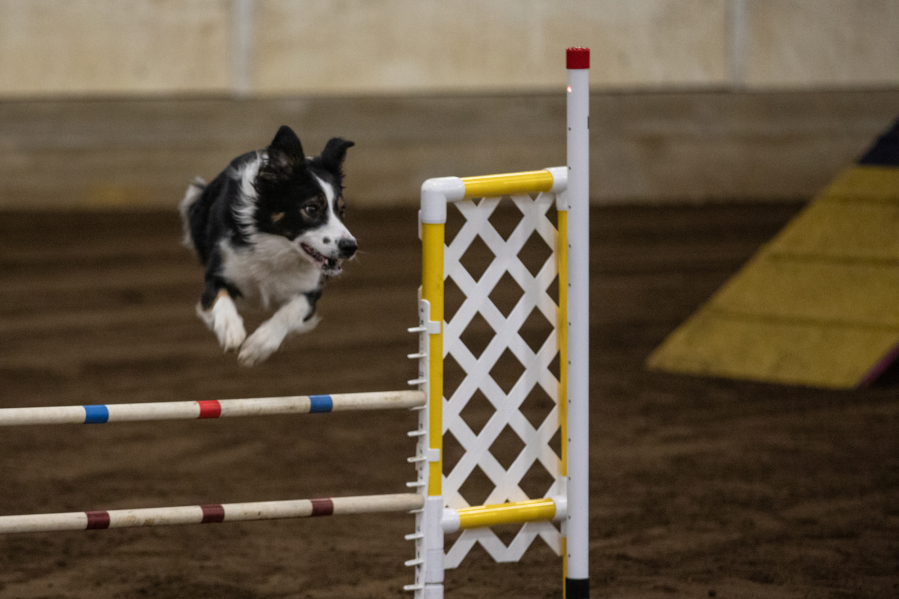The image captures a lively black and white Border Collie participating in an agility competition. The photograph is taken from the front, showing the dog in mid-air as it jumps over a set of two horizontal poles. The dog's ears are perked up, and it appears to be looking slightly to the right, possibly at its trainer. The top pole is made of wood and features blue-red-blue stripes, while the bottom pole is a white rod adorned with three brown stripes. Supporting these poles is a structure made from white and yellow PVC piping with white netting. To the right of the dog is a small plastic fence in white and yellow with a red top and a yellow ramp, likely part of the agility course. The background is blurry, suggesting an indoor setting, and the ground appears to be made of dirt, providing a safe landing surface for the dog.